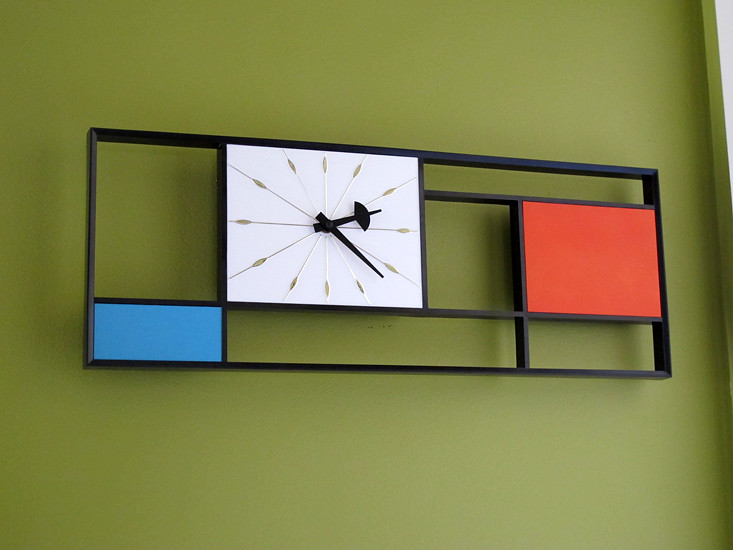In the image, there is a uniquely designed clock mounted on a green wall. The clock itself is rectangular in shape and crafted from black metal. The design features an artistic composition of three rectangles: a blue rectangle at the bottom, a red rectangle slightly above and to the right, and finally, in the center, a white square housing the clock face. 

The clock's face is adorned with black hour and minute hands, showing the time at 2:22. Radiating outward from the central clock face are numerous gold lines, each strategically positioned to represent one of the twelve hours on the clock. These gold lines give the appearance of a radiant sunburst, adding an element of elegance and visual interest to the piece.